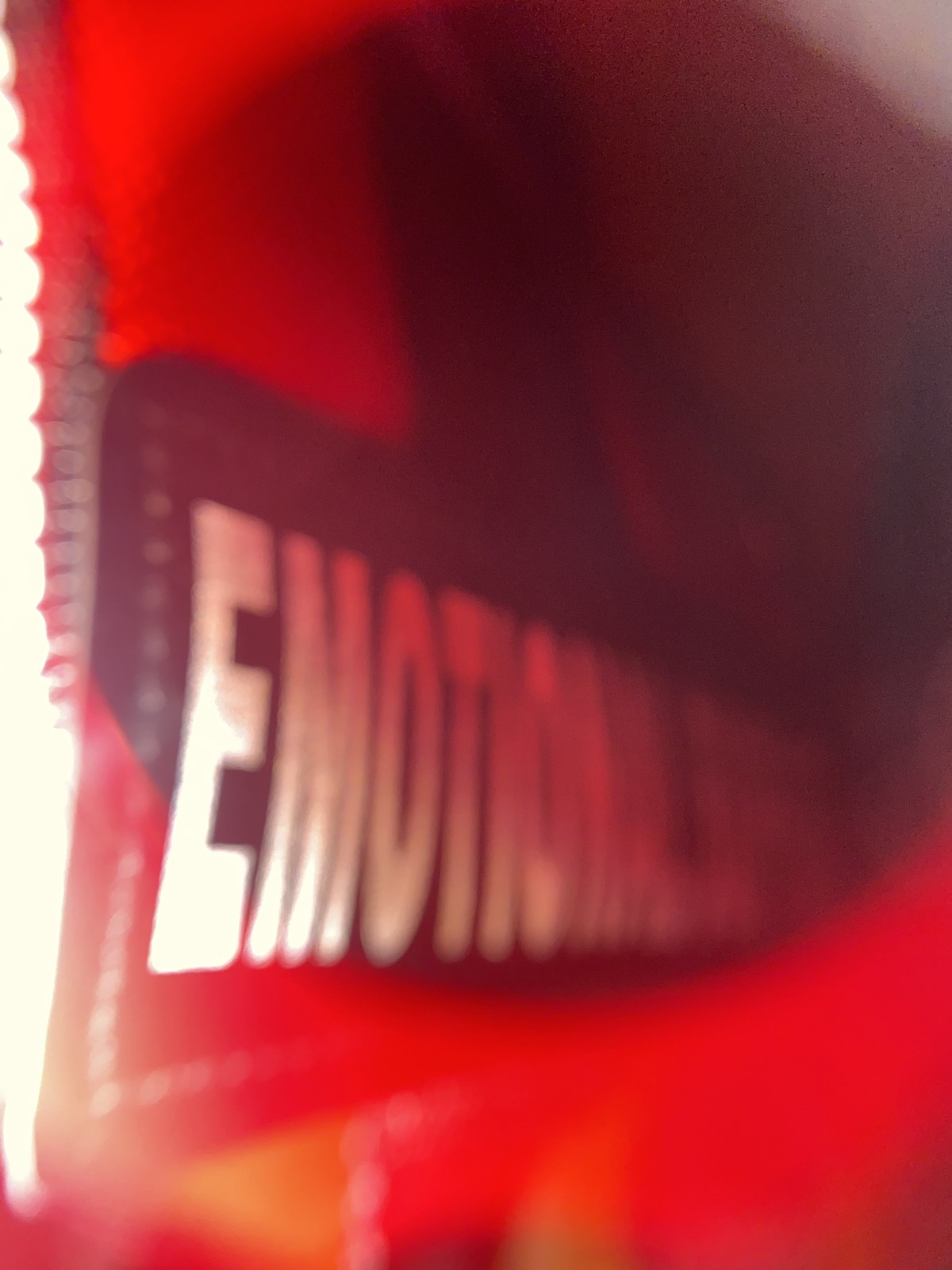A vertical, vibrant red image that could be a photograph or a digital rendition. The composition is dominated by varying shades of red, creating a rich, textured backdrop. A strip of black floats through the image on a diagonal axis, featuring partially obscured white text that leans askew, reminiscent of a sign viewed from an angle. The visible portion of the text reads "emotional," hinting at additional words that are cut off due to the angle. The interplay of colors and text creates a dynamic and somewhat enigmatic visual effect.